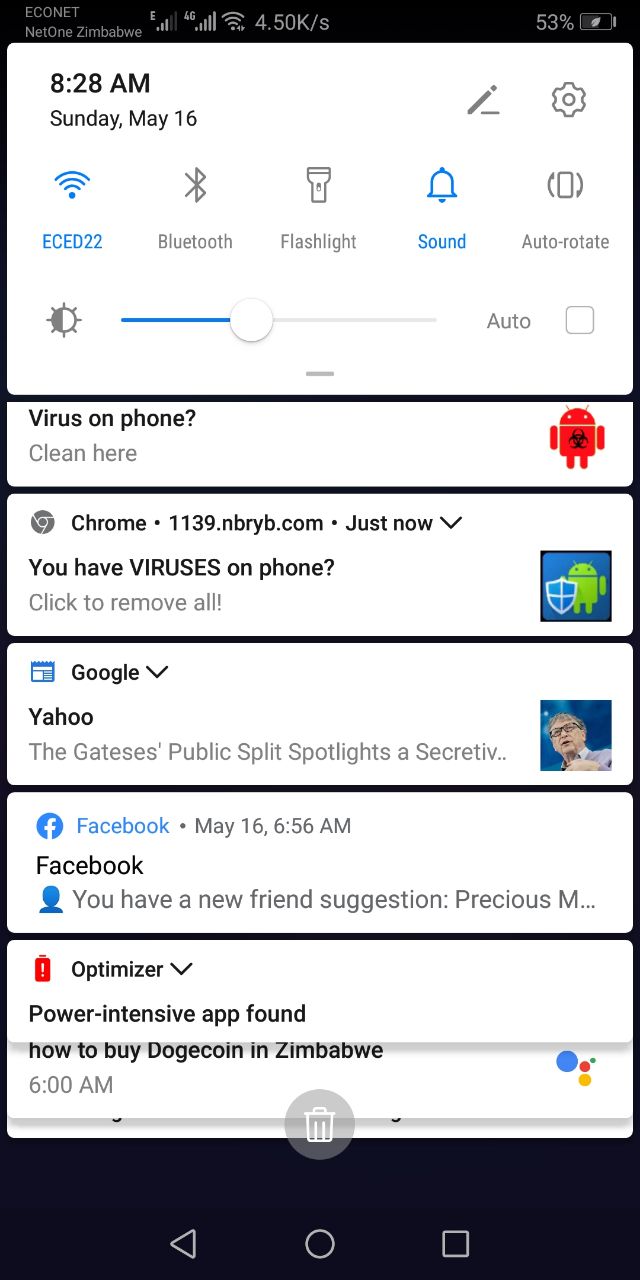This screenshot, taken at 8:28 AM on Sunday, May 16th, captures the Android Notification Shade on a device connected to Econet Zimbabwe with 4G LTE. The status bar indicates the battery level is at 53%. Various notifications are visible:

- A virus warning from Chrome, originating from 1139.ryb.com, advising the user to clean their phone, which is identified as a potential threat.
- A Google News update about the Gates Public Split, sourced from Yahoo!.
- A Facebook notification suggesting a new friend, with the name beginning with Precious.
- An optimizer alert identifying a power-intensive app.
- A Google Alert reminder regarding how to buy Dogecoin in Zimbabwe, received at 6:00 AM.

The quick settings panel appears at the top, featuring toggles for WiFi, Bluetooth, flashlight, sound, and auto-rotate. The brightness slider is set slightly below medium.